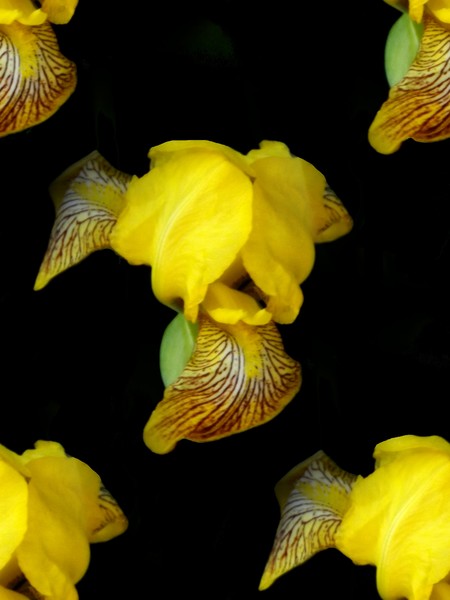This image displays five yellow flowers, resembling irises, against a black background. The focal point is the central flower, showcasing a mix of partially bloomed petals: some bright yellow and others adorned with intricate brown veins. The top petals fan outwards, displaying a blend of white and yellow with prominent veining, while the bottom presents a triangular-shaped petal with similar coloring. Around the central flower, each corner of the image features a partial illustration of additional irises. The petals in the corners exhibit curved forms, with the upper ones primarily revealing the interior, vein-lined surfaces, and the lower ones showing predominantly bright yellow petals. A touch of green, possibly a leaf or bulb, is visible at the bottom left. The lack of visible stems accentuates the flowers' vivid yellow and brown hues against the stark black backdrop.